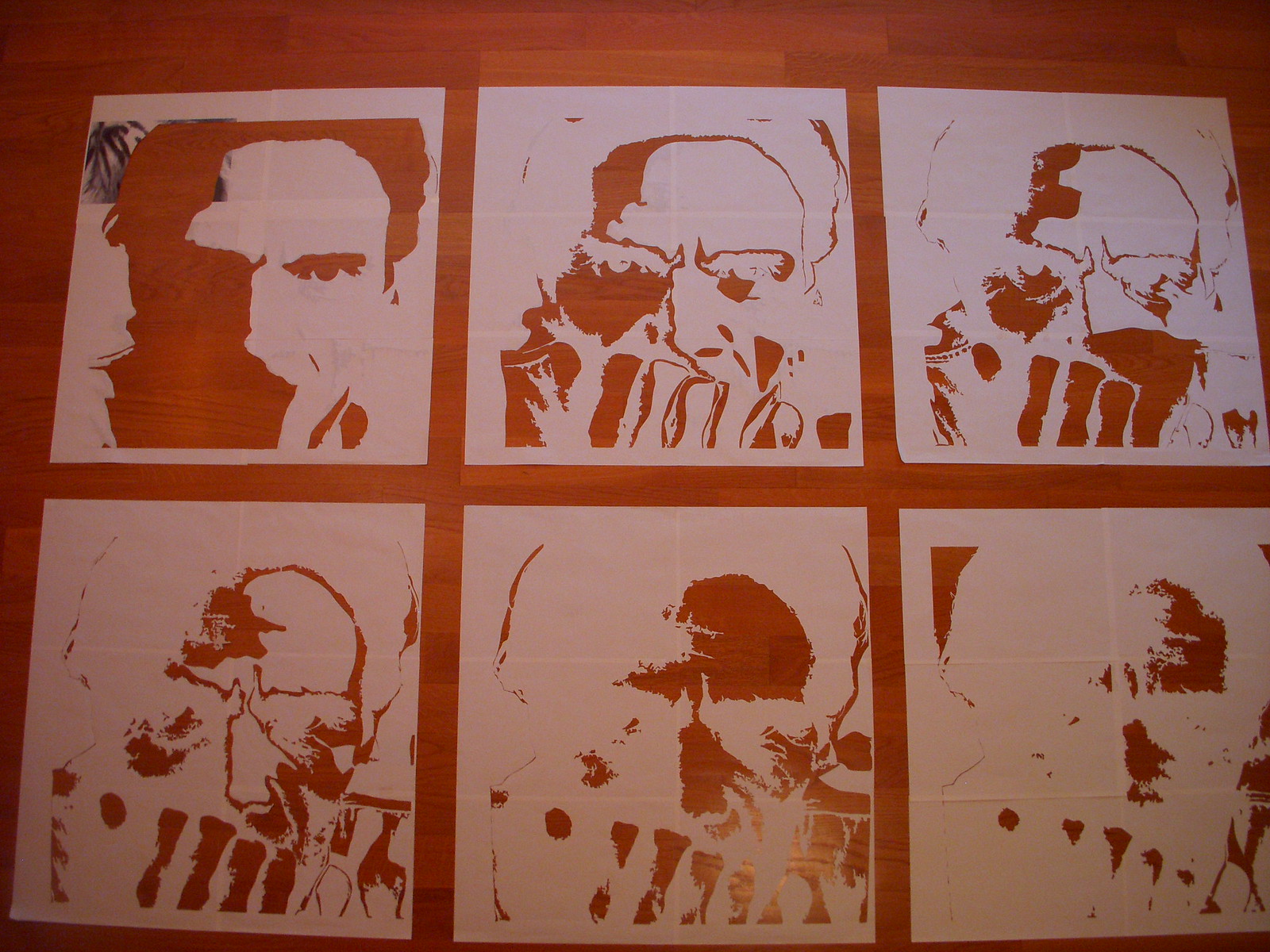The photograph displays six distinct stencil art pieces, each portraying the same face but with varying levels of detail and exposure, creating an illusion of different faces. These stencils are arranged in two rows of three on a light wooden laminate floor, which frames the artwork. Each white square features cutouts that reveal the brown wooden surface beneath, enhancing the contrast and adding depth.

In the top left, the stencil reveals a distinctly dark image, predominantly shadowed on the left side but with a visible eye on the right. The top center image presents the face with more defined eyebrows, giving a stark contrast between the whitened brows and the darkened eyes. The top right piece shifts focus to the right side of the face, partially obscuring the left side.

On the bottom row, the left stencil mirrors the top right but begins to fade in color. The bottom center piece further fades, with noticeable darkness only around the forehead and nose areas, suggesting an overexposed effect. Finally, the bottom right image is profoundly overexposed, revealing almost no discernible details.

Throughout all images, the recurring outlines and gradual overexposure emphasize the transformative effect, moving from clarity to abstraction. This sequence not only highlights the artist's technique in using stencils but also invites viewers to observe the progressive loss of detail and the conceptual metamorphosis of a single face.